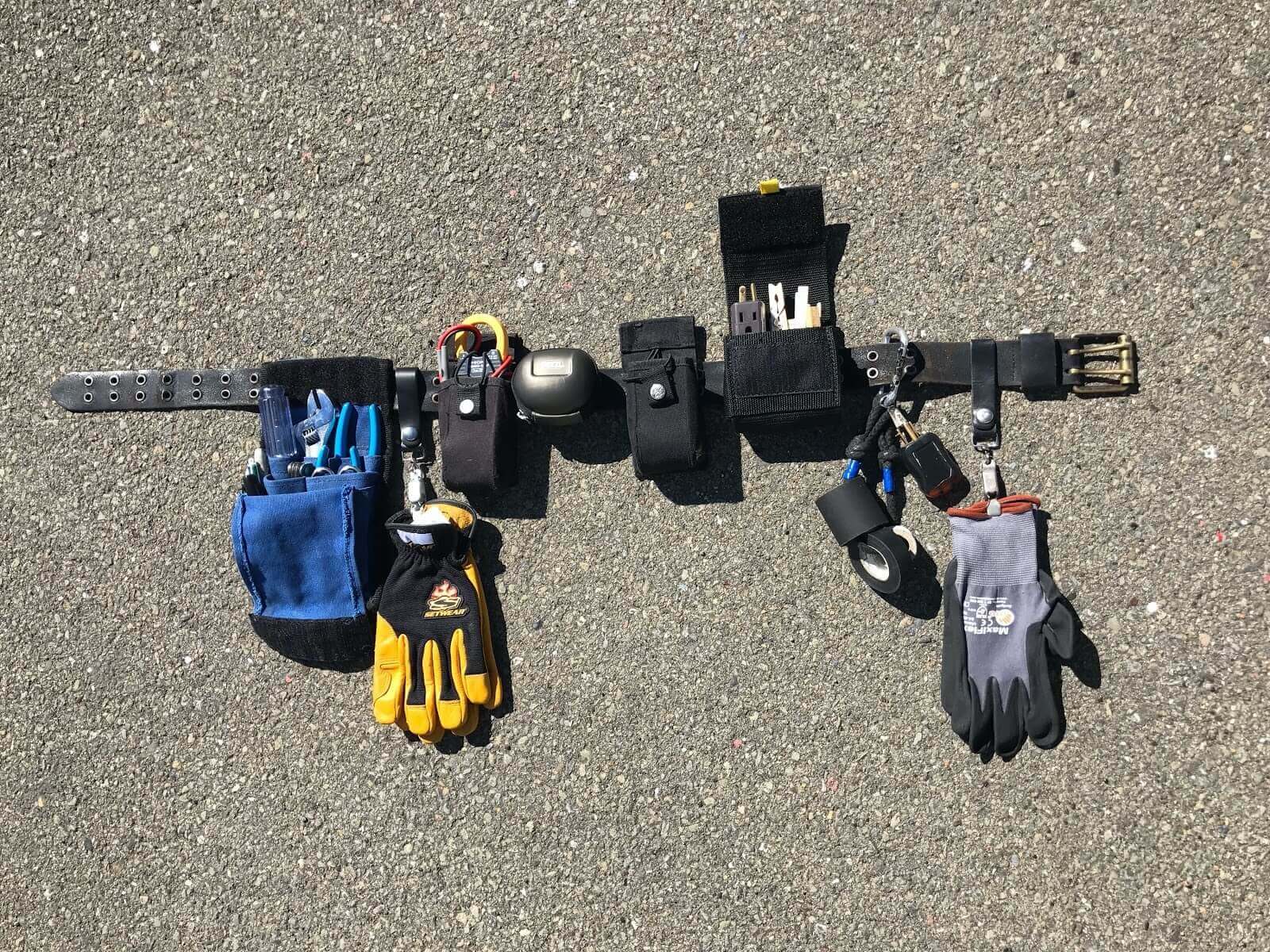This image portrays a meticulously organized black utility belt laid out on a gray gravel surface, resembling pavement. The belt features a gold buckle on the right and double notches running along the left side. Various tools and items are attached to it, suggesting it belongs to a maintenance worker. Moving from right to left, the belt includes: a pair of gloves with yellow tips, a roll of duct tape, a carrying case holding an electrical outlet and metal pieces, a knife case, a black oval gauge, some wires, another set of gloves with orange accents, and a blue multi-tiered fabric sack containing tools like screwdrivers and a wrench with blue handles. These items are precisely arranged, indicating the utility and preparedness essential for the belt's user.